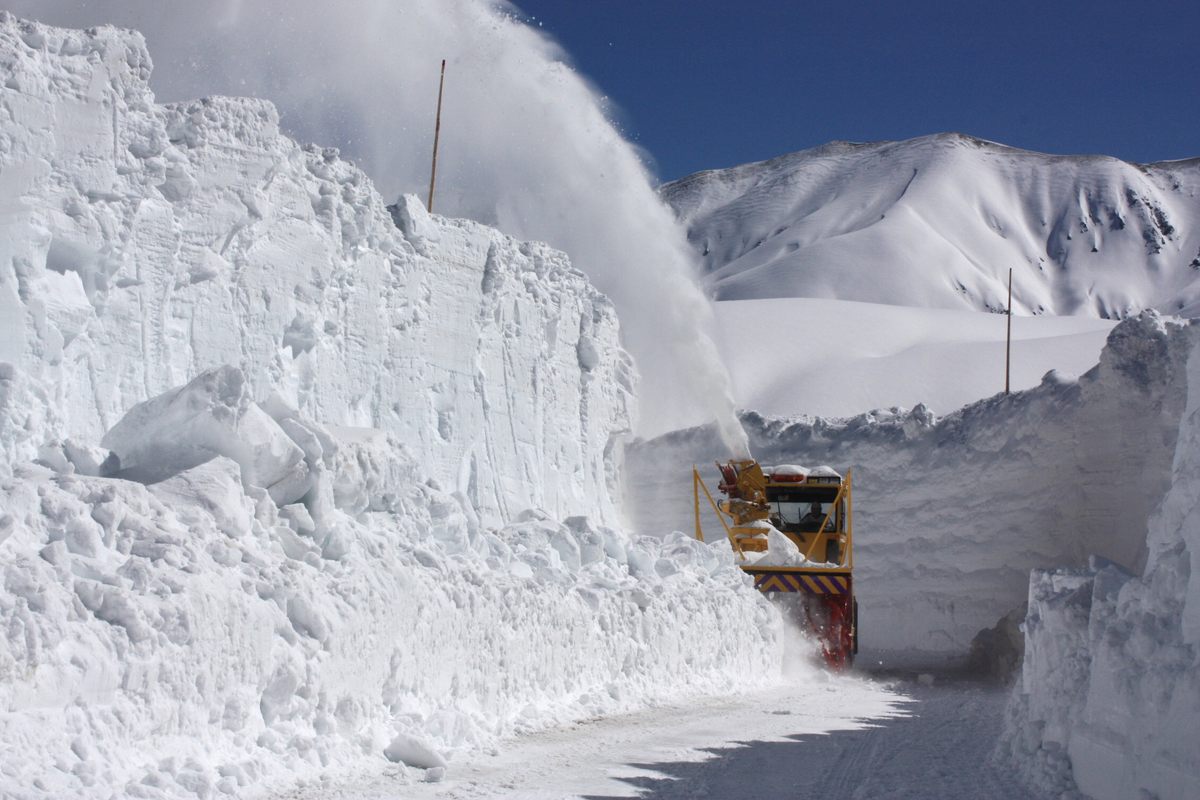In this outdoor image, a massive rotary snow plow is actively clearing a snow-covered mountain road. The towering mounds of snow, which reach up to the height of a one-story building or about 15 to 16 feet, dwarf the already tall yellow machine with red wheels. The snow plow is efficiently sucking in the immense snowdrifts and shooting the snow up and out to the sides, creating a narrow path through the thick snow embankments. The sky above is a clear blue, with a rugged, snow-laden mountain standing majestically in the background. Telephone poles along the road are nearly buried, with only about four to five feet visible above the deep snow. The scene is one of sheer winter intensity, capturing the essence of a high-altitude area blanketed in heavy snowfall. Shadows and holes in the snow add depth to the scene, emphasizing the arduous task of keeping the road navigable.